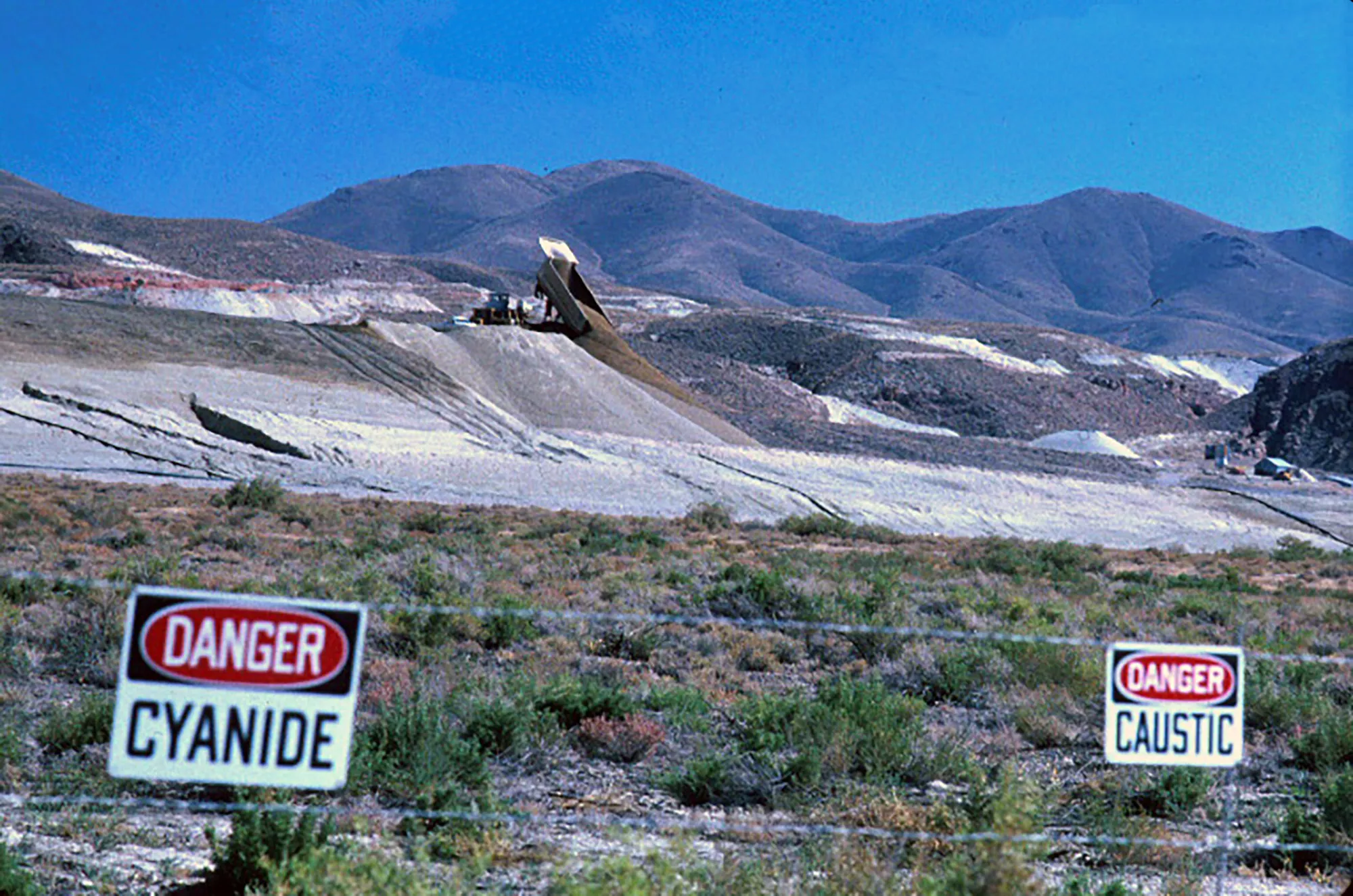In this stark and desolate landscape, a barren hillside is juxtaposed against a backdrop of bare, lifeless mountains under a blue, cloudless sky. The foreground is dominated by a dusty, desert-like field, where a dump truck is actively offloading more material onto a large pile of dirt, its front facing left and the bed elevated. The scene is fenced off with a double line of silver barbed wire, adorned with ominous signs. On the left, a black-topped sign features the red, bold warning "DANGER" with "Cyanide" written below in black lettering, while a matching sign on the right warns of "Caustic" in the same stark formatting. Patches of white, possibly chemical residues, litter the area, enhancing the perception of a hazardous dump site. The mountains in the backdrop lack any visible trees, wildlife, or water, emphasizing the aridness and inhospitable nature of the environment. The relentless sun beats down on the scene, intensifying the sense of desolation and danger.